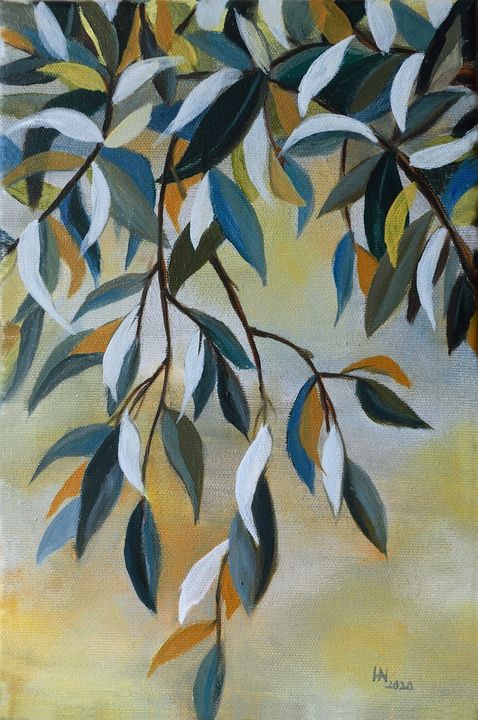This artwork depicts an ethereal hanging foliage scene, where slender branches cascade downwards from the top of the canvas. The background is a seamless melding of shades—grey, white, pale orange, and pale yellow—creating a softly smudged, almost ethereal backdrop. The main focus is the delicate leaves, which grow from thin stalks and are connected by even finer offshoots. These leaves are masterfully painted in a spectrum of hues including light blue, orange, black, dark grey, teal, and sage, with some blending into mixed shades. The density of the foliage is most concentrated at the top, representing the proximity to the tree's main body. As the branches extend downward, they progressively thin out until a singular branch reaches the image's lower bounds, where the leaves transition into shades of white, orange, and blue. This detailed interplay of colors and structure gives the artwork a serene and organic complexity, capturing the viewer's eye with its intricate and graceful depiction of nature.